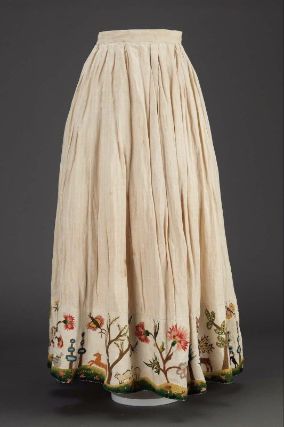This is a photograph of a long, cream-colored skirt displayed on a white stand against a dark grey background. The image is oriented vertically, accentuating the full length of the garment, which nearly reaches the floor. The skirt appears to be made from a soft fabric, possibly linen or cotton, and is designed with a heavily pleated or gathered waistband, giving it ample movement. The bottom of the skirt features an intricate embroidered border with dark red and dark pink flowers, dark stems, and additional motifs such as butterflies, trees, small horses, and sheep, all set against a backdrop of grass. Beneath this detailed stitch work is a black border running along the very edge of the hem, contrasting with the cream fabric and adding a final touch of elegance to the piece.